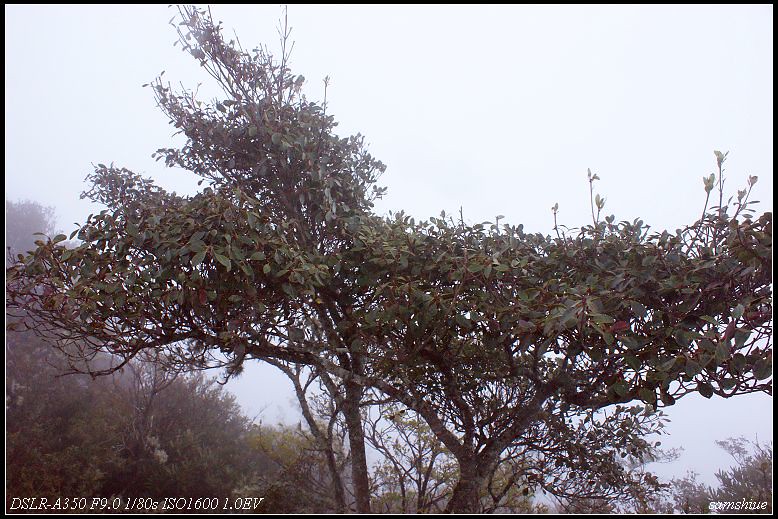The image captures a foggy scene with a dominant, hazy white sky overhead. Stretching from almost the top center of the frame is the crown of an expansive tree, filled with branches adorned with green leaves, some showing hints of red and yellow, suggesting the early stages of seasonal change. The tree dips slightly in the center, but its foliage spreads widely across the image. Below this, the sturdy brown trunk and branches are visible, emphasizing the tree's impressive stature. The background fades into a distant, blurry collection of greenish trees, partially obscured by the fog. In the bottom right corner, technical details about the photograph are noted: "DSLR, F 9.0, 1/80 seconds, ISO 16001.OEV." This comprehensive setting adds context to the ethereal and serene landscape.